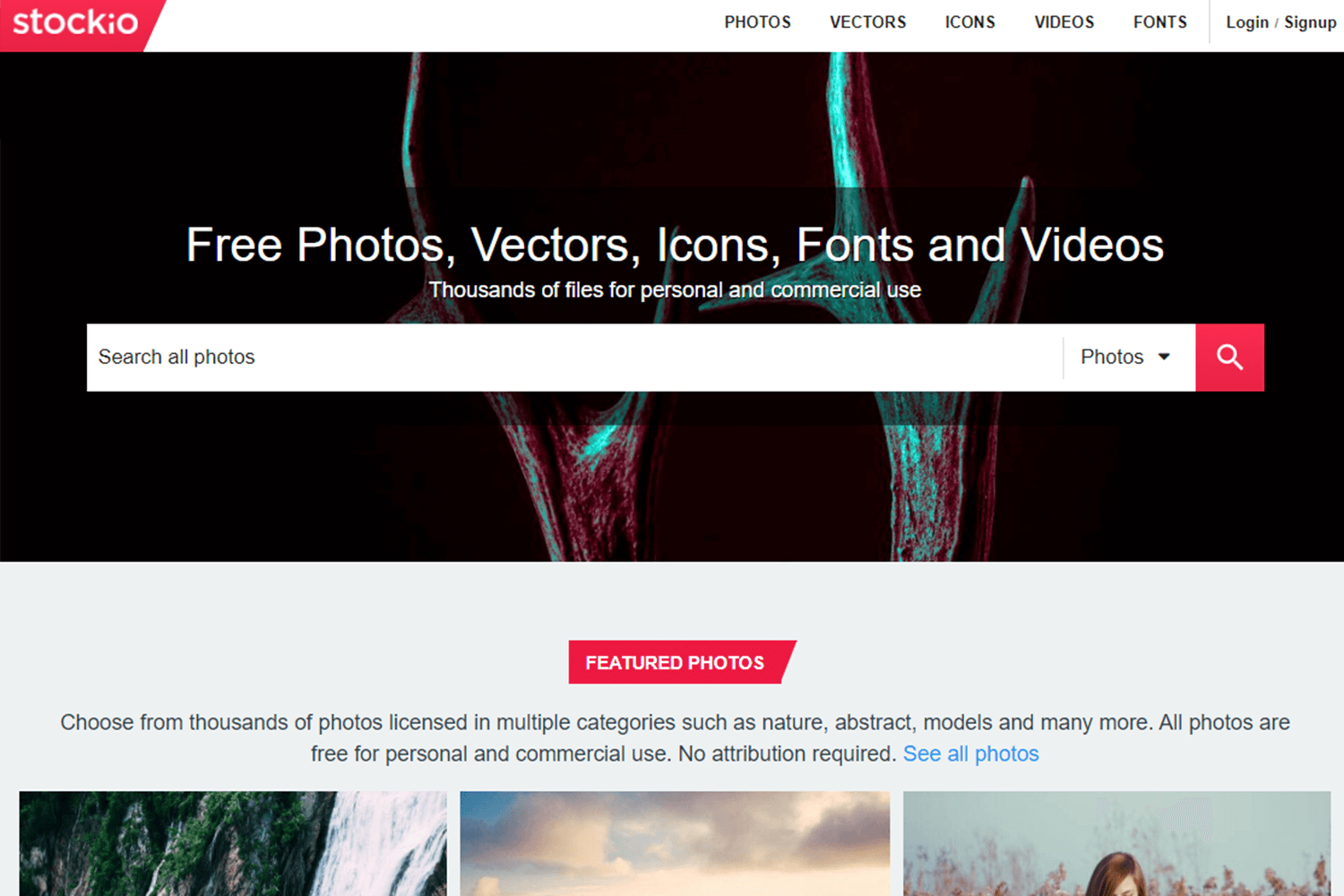This screenshot captures the homepage of a website called Stockio. The name "Stockio" is prominently displayed in white text within a red box. The navigation bar at the top offers several options: Photos, Vectors, Icons, Videos, and Fonts, along with login and sign-up links. Just beneath the navigation bar, the text "Free photos, vectors, icons, fonts, and videos" emphasizes that thousands of files are available for both personal and commercial use. There's a search bar centrally located, accented with a red box around the magnifying glass icon, allowing users to search for specific media.

Below the search bar, the site highlights "Featured Photos" in white text within another red square. Three sample images are displayed: the first image has a dark background with what looks like antlers and gradient 3D colors; the second image features a city skyline; and the third image showcases a waterfall. Users can also click a blue link labeled "See all photos" to explore more options.